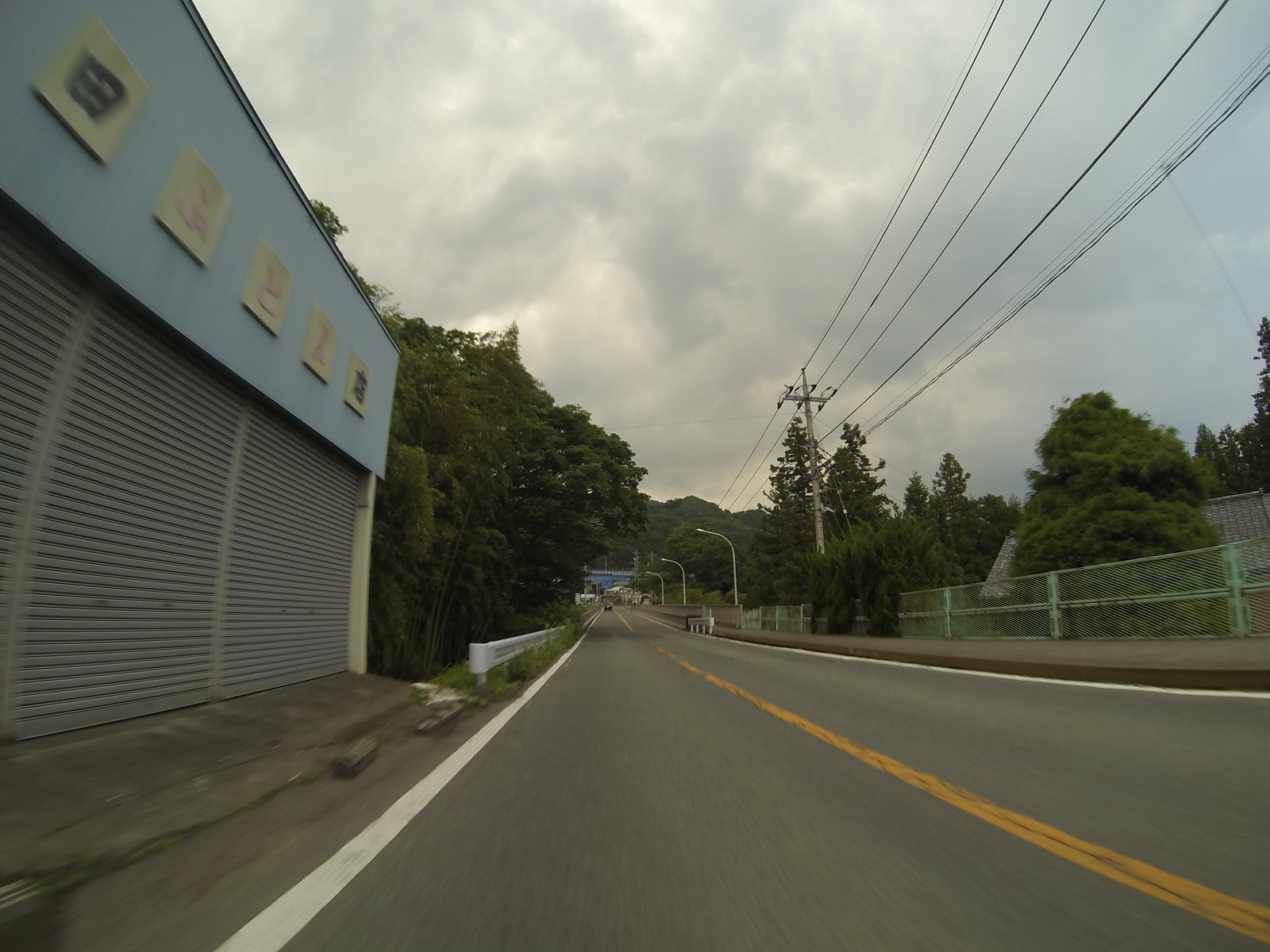A downward view of a street features a row of three garage doors on the left side, two of which are fully visible while the third is partially seen. Above the garage doors, the wall is painted blue and adorned with various white advertisements. The road extending in the image is long, with the garage doors positioned very close to it. Adjacent to the garage doors on the left, a guardrail runs parallel to the road. On the right side, there's a sidewalk bordered by a fence, and a series of utility poles stretch along the street with cables running between them. Further down the road, streetlights begin to appear, arching over the roadway. Trees line the left side of the street and are also visible in the distance on the right and far down the road. The sky is overcast, adding a cloudy backdrop to the scene.